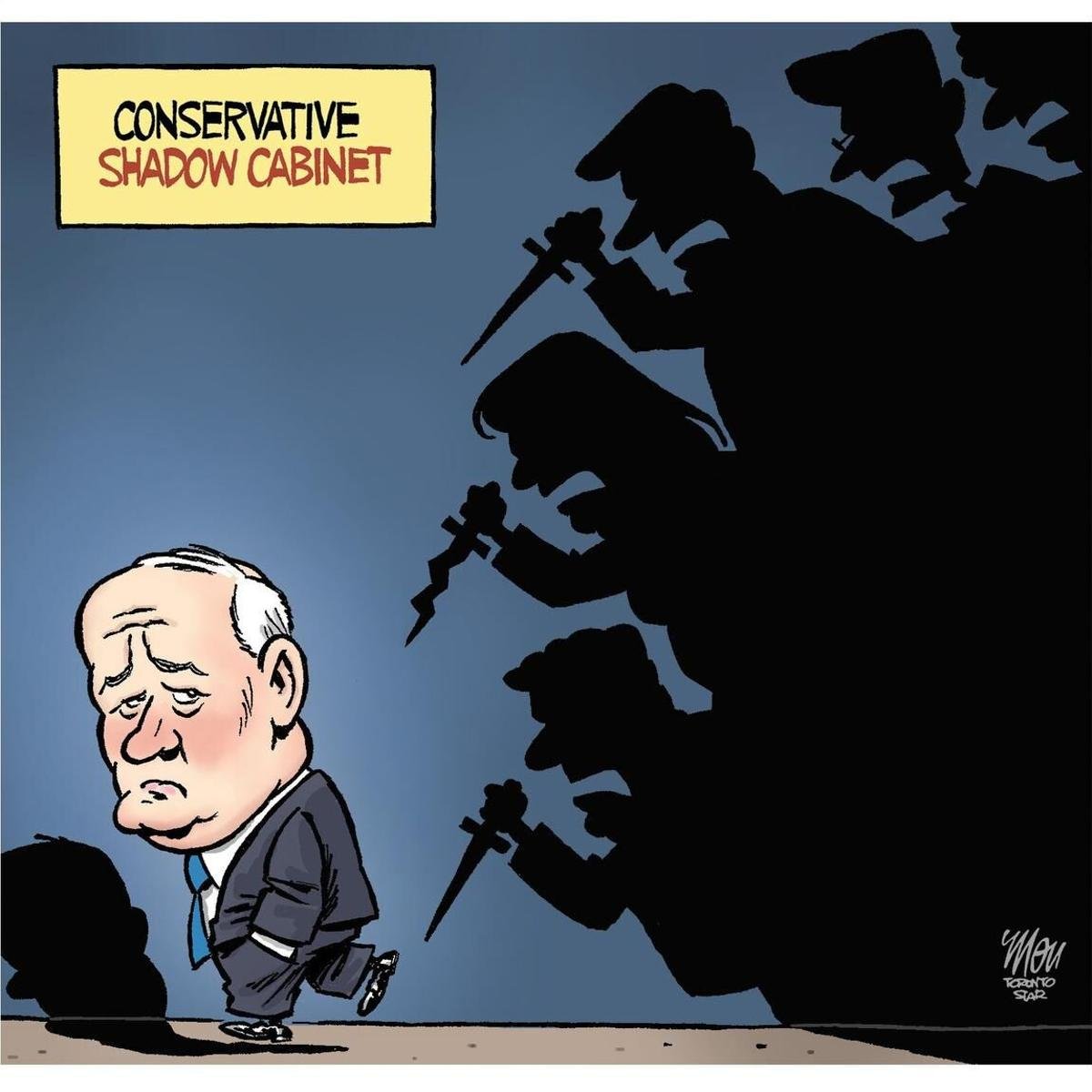In this detailed political cartoon, a short, heavyset older man with a disproportionately large head, white receding hair, worried eyebrows, and a protruding chin, dressed in a blue jacket, bright blue tie, white shirt, black shoes, and black boots, is walking away with a sorrowful expression. He is positioned on the bottom left side of the image, with his shadow cast against a solid grey-blue background and a grey floor. This background is topped with a yellow rectangle framing red and black text which reads "Conservative Shadow Cabinet." Looming behind the man to his right, an intimidating tower of dark, shadowy figures wielding various sharp weapons, including daggers and swiggly knives, points their blades menacingly downward towards him. These shadowy characters have their mouths open as if shouting angrily, adding to the man’s evident distress. The overall tone of the cartoon is dark and foreboding, reflecting political tension and opposition.